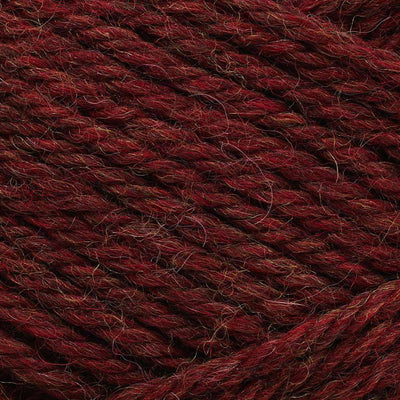The image is a close-up of a tightly rolled spool of red yarn, characterized by its deep, almost burgundy hue. The yarn is uniformly wound in a precise manner, creating a neat and organized appearance, although there are a few loose strands and slightly fuzzy fibers visible. The texture suggests a standard width yarn, intended for knitting. The image is uniformly dedicated to showcasing the yarn without any additional background or text. The right bottom corner of the image hints at a different pattern or direction in the yarn's texture, adding a subtle complexity to the otherwise singular display.